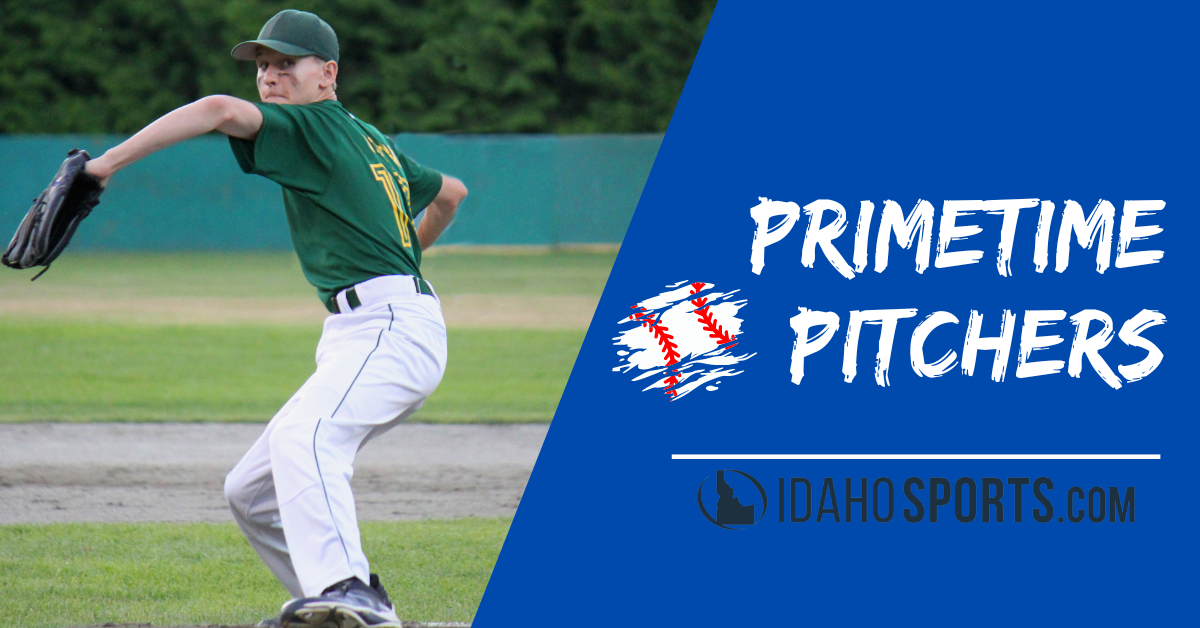The horizontally aligned rectangular image is divided into two distinct trapezoidal sections. The left half features a vibrant baseball field with a dense, blurry line of green trees in the background, topped by a solid green wall. The field itself displays shades of green and brown. Dominating this section is a thin baseball player captured in a side view mid-throw. He wears a green and yellow jersey, white baseball pants, a green baseball cap, and holds a black glove on his left hand. On the right half, the image transitions into a solid bright blue background. In its center, bold white capital letters spell out "PRIMETIME PICTURES," accompanied by an artistic rendering of a jagged-edged baseball. Below this, a white line runs horizontally with "IdahoSports.com" presented in black capital letters beneath it. The overall image is brightly lit and meticulously clear, emphasizing the dynamic action of the pitcher against the contrasting promotional design.